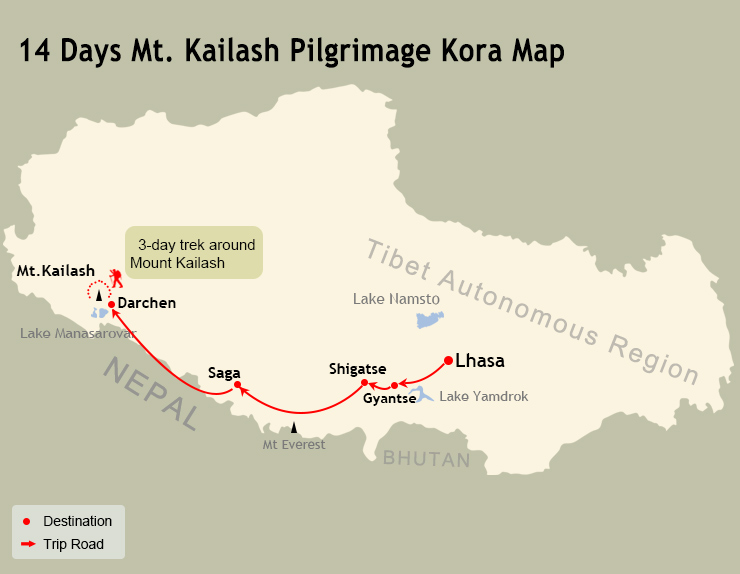This image is a detailed map titled "14 Days Mount Kailash Pilgrimage Korra Map," set against a light brown or khaki-colored background. The central focus of the beige map area is the Tibet Autonomous Region, with Nepal and Bhutan marked towards the bottom. Notably, it highlights a three-day trek around Mount Kailash, depicted by a tiny black triangle with a red dotted line encircling it.

The route starts from Lhasa, progressing through Gyantse, Shigatse, Saga, and ending in Darchen, marked by red dots connected by red arrows. Each trekking point is annotated with its name for clarity. A red silhouette of a hiking figure is shown at the end of the route near Mount Kailash, denoted in a box that reads "three-day trek around Mount Kailash."

Additionally, the map features a gray box at the bottom labeled with a red dot that says "Destination" and a red arrow indicating "Trip Road." This meticulously planned route offers a clear guide for pilgrims and backpackers, providing a sense of the journey and the key stops along the way.